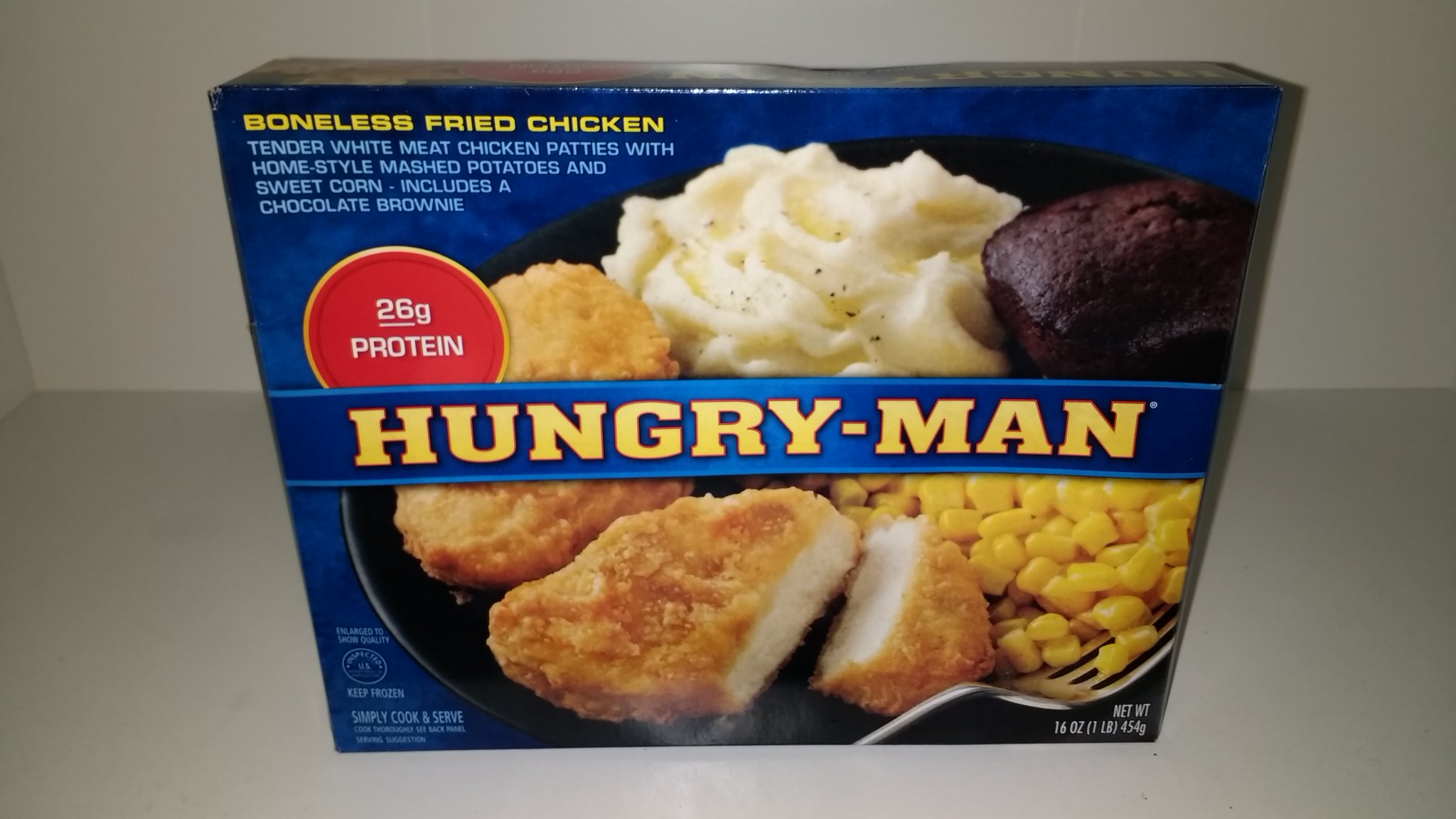The image displays a Hungryman microwavable TV dinner featuring boneless fried chicken. The box contains tender white meat chicken patties, homestyle mashed potatoes, sweet corn, and a chocolate brownie. The packaging is primarily brown, with the product prominently seated on a white shelf against a white background. The brand name "Hungryman" is clearly visible in large, bold yellow letters on the front of the box. The front of the packaging also showcases a detailed picture of the meal, highlighting the mashed potatoes, chicken nuggets, corn, and brownie. A striking red sticker on the front indicates that the meal contains 26 grams of protein.